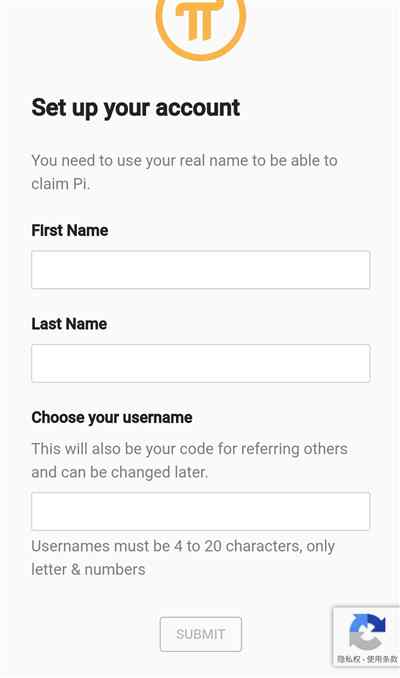The image features a user interface on a white background. At the top of the interface, there is an orange circular symbol with a white interior, though the top part of the circle is cut off. This symbol includes a horizontal orange line intersecting two parallel vertical orange lines.

Below the symbol, "Set up your account" is prominently displayed in black text. Beneath this heading, in gray text, it states, "You need to use your real name to be able to claim a PI."

The form begins with fields for "First Name" and "Last Name," each labeled in black text, and accompanied by white data fields bordered in gray. Following these fields, there is a section labeled "Choose your username" in black text, with an additional note in gray below: "This will be your code for referring others and can be changed later." The corresponding username data field is also white with a gray outline and contains a gray placeholder text instructing that "Usernames must be four to twenty characters, only letters and numbers."

At the bottom right of the form, there is a CAPTCHA with a gray outline and a white interior. The CAPTCHA features an arrow that starts on the right and curves to the left, transitioning in color from gray to light blue to dark blue, and topped with smaller arrows. Below the CAPTCHA, there appears to be text that is blurry and seems to be written in kanji.

Finally, there is a "Submit" button outlined in gray with "SUBMIT" in capital letters written in gray.